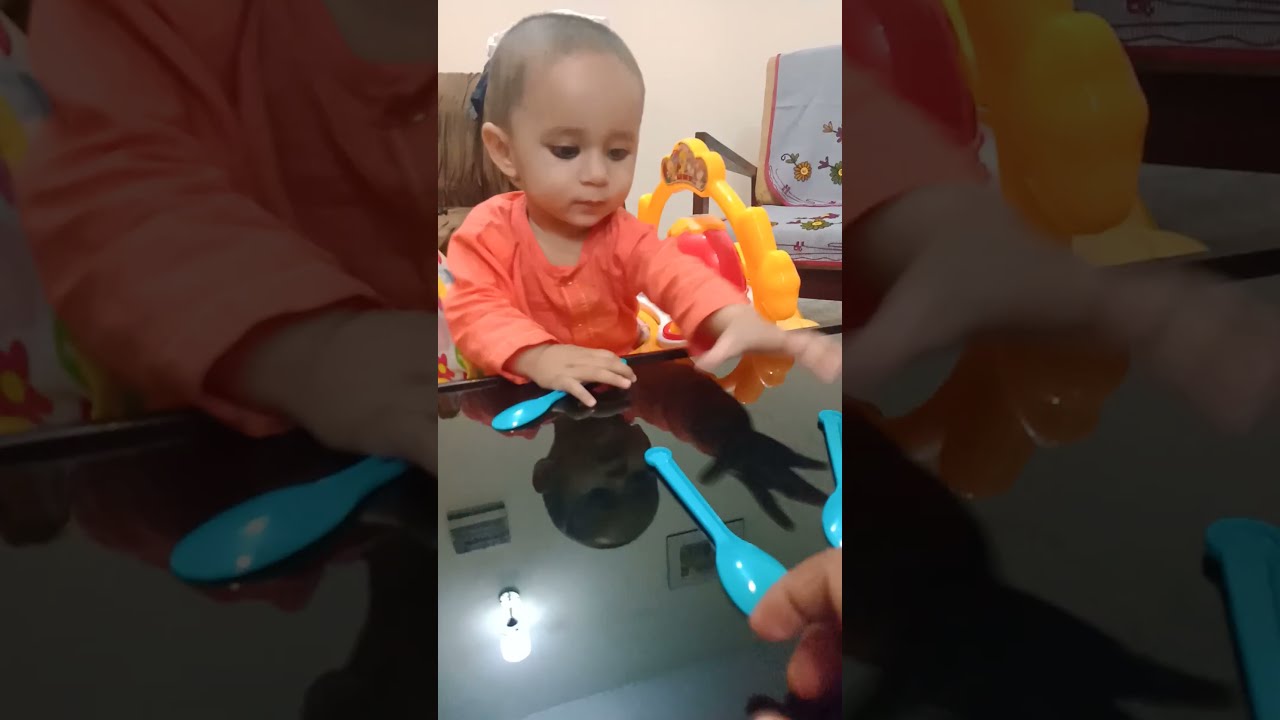The image features a young child, possibly of Indian descent, whose gender is somewhat ambiguous but possibly a little girl based on facial features. The child, who appears almost bald with very short, thin hair, is centered in the view and wearing an orange or peach-ish pink shirt. She is seated at a black, reflective table, reaching out with her left hand to grab a blue spoon, while already holding another blue spoon in her right hand. 

In front of the child, there are more blue spoons scattered on the table, and the fingers of an adult can be seen in the bottom right corner, suggesting interaction or play. Behind the child, there are various toys, including a notable yellow toy with crown-like spikes and an orange seat. Also visible are two sofas, a darker brown one with a blue drape and a lighter brown one, set against a yellowish wall that transitions to white. This indoor setting is bathed in a mix of colors like orange, yellow, brown, green, and light blue. Additionally, there is a large, reflective black monitor or TV screen in the background, topped with more blue plastic toys, contributing to the overall playful and engaging scene.